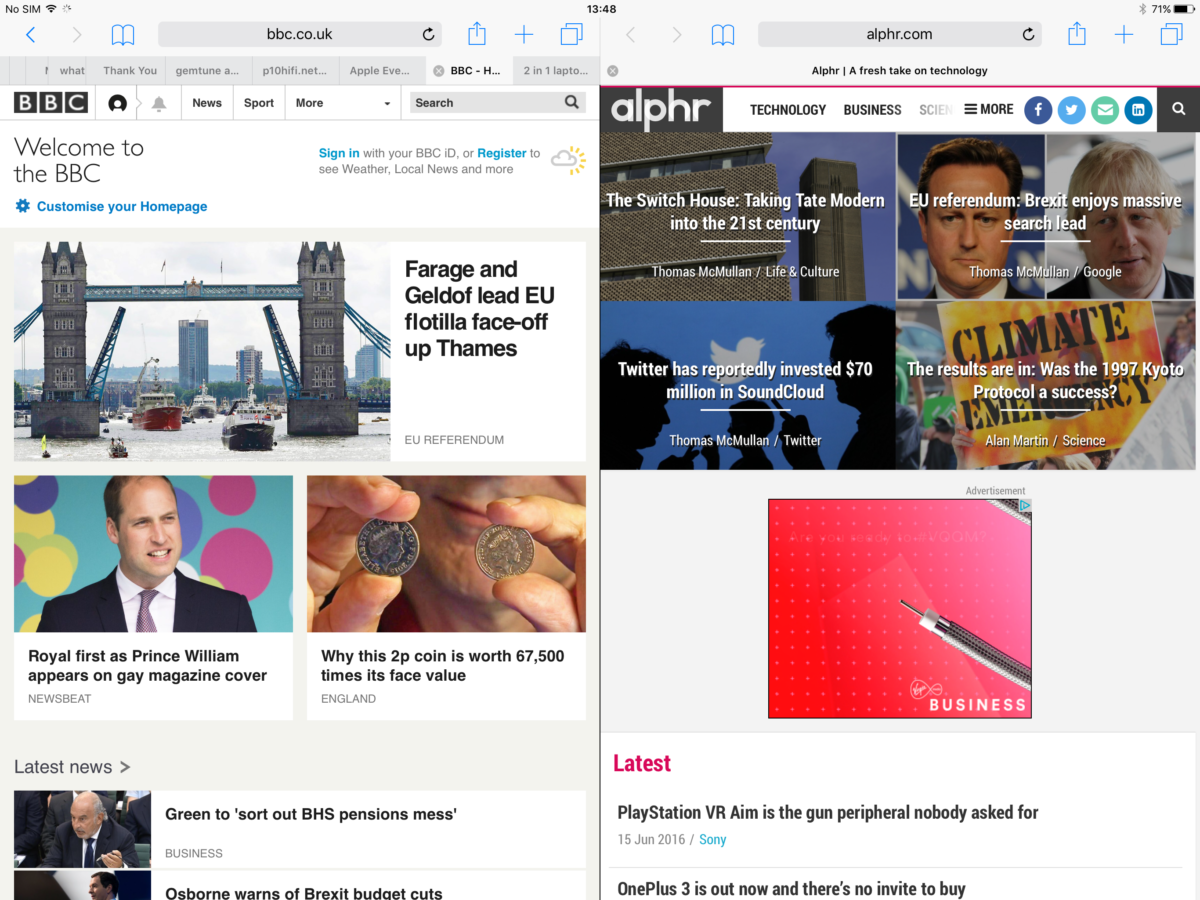A detailed caption based on the given voice input could be:

"An image of Nelson featuring prominently, symbolizing connectivity and access to information. The visual elements suggest themes related to Wi-Fi networks and online platforms such as BBC.co.uk, highlighting Nelson's association with modern technology and media."